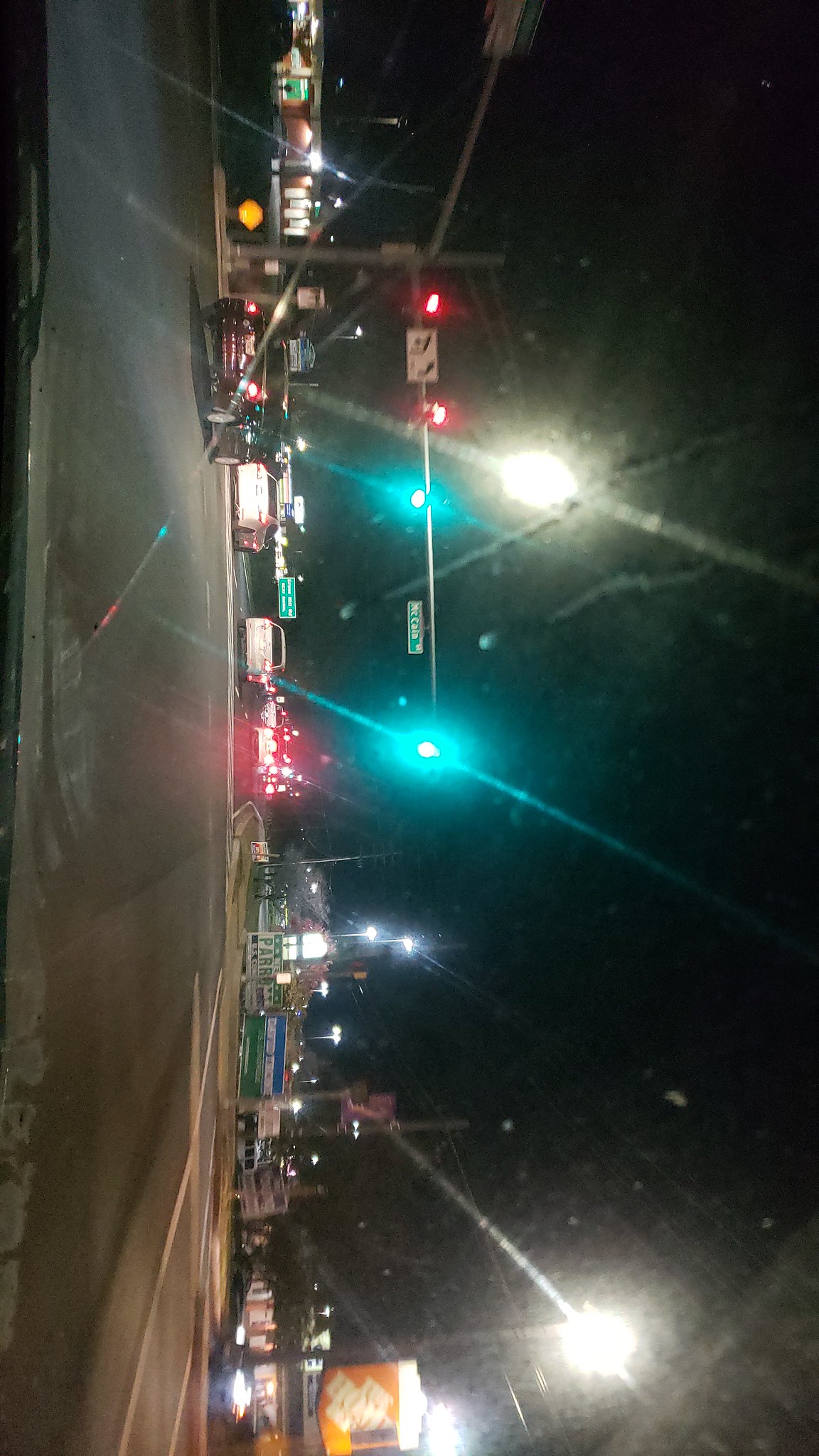A tilted portrait photo captures a bustling streetscape at night, erroneously displayed in landscape orientation. The rectangular image, viewed sideways, presents an urban scene illuminated by various lights. Dominating the central composition are two green traffic lights, positioned slightly below two red lights. Below these signals, several cars are depicted either stationary or in motion, their headlights piercing the night. Evidence suggests the photo was taken from inside a vehicle, as a windshield wiper is visible in the upper left corner. The street is flanked by businesses, including a distinct orange sign at the bottom, identifiable as a Home Depot sign. The background is dotted with additional business lights, and green street signs are suspended in the center, contributing to the urban nighttime atmosphere.